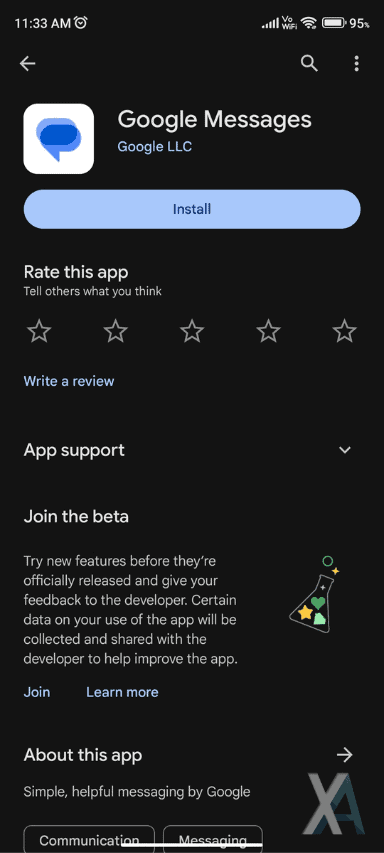The image showcases a smartphone screen displaying the Google Play Store page for the "Google Messages" app. At the top of the screen, there are standard status bar details including the time, battery percentage, and WiFi signal strength. Below that, navigation icons such as a back arrow, a white magnifying glass, and three vertical white dots are visible.

The central part of the screen prominently features the app's name, "Google Messages," with a background showing a blue messaging bubble and labeled "Google LLC." Beneath this section, there is a blue "Install" button allowing users to download the app.

Further down, users are prompted to rate the app, with a five-star rating system and a blue "Write a review" button. There is also an expandable "App support" section, marked by a downward-facing arrow.

Additionally, the screen provides an option to "Join the beta," inviting users to try new features before their official release and give feedback to the developer. The text underlines that some usage data will be collected and shared with the developer to improve the app. This section includes blue "Join" and "Learn more" buttons, along with an icon resembling a flask adorned with a green heart, yellow star, and green section, symbolizing a science experiment or beta testing.

Near the bottom, there is an "About this app" section that states, "Simple, helpful messaging by Google," classified under "Communication" and "Messaging." An icon labeled "XA" appears with the 'X' in gray and 'A' in green, although its specific purpose is not clearly described in the text.